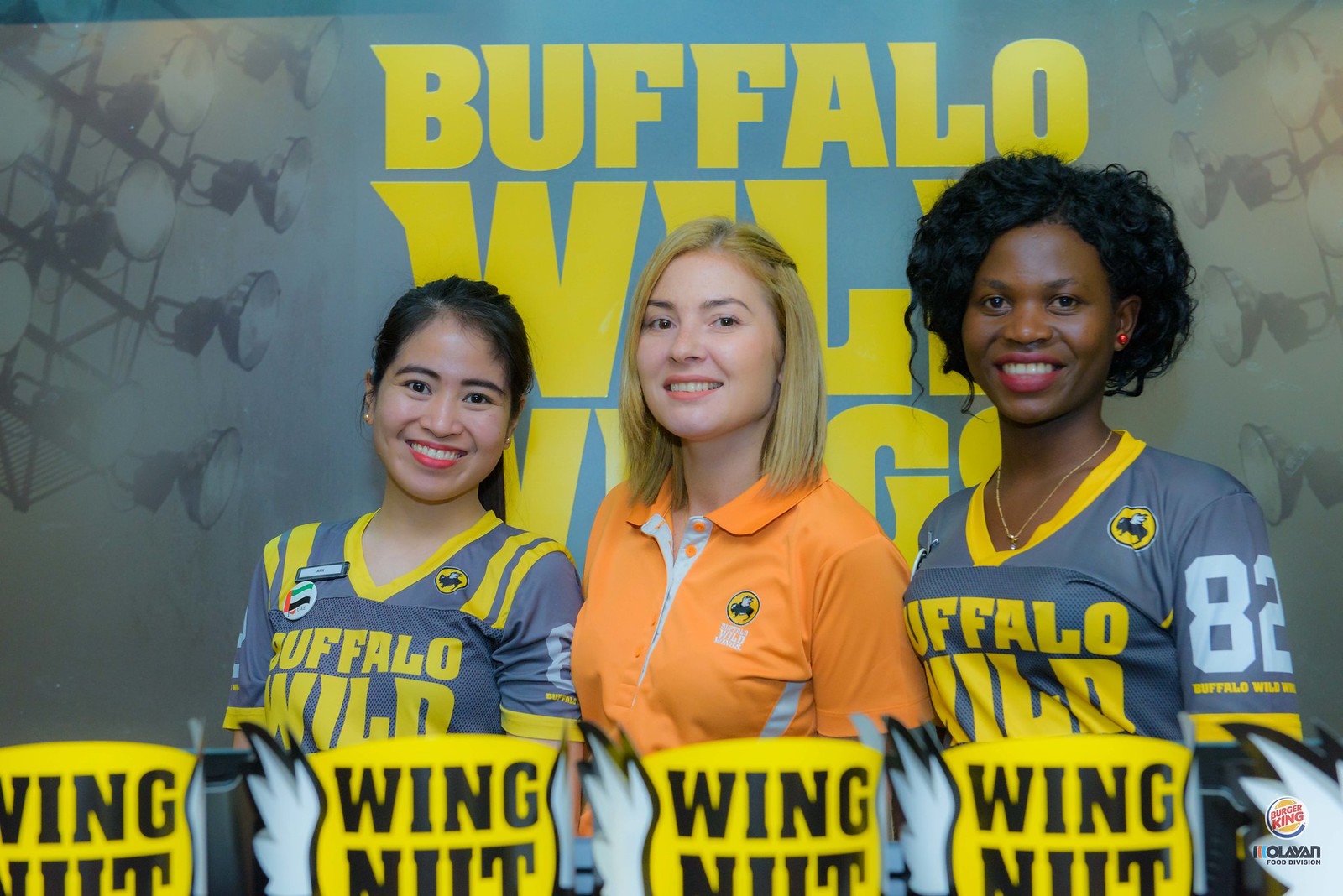This photograph captures three smiling women against a grey backdrop adorned with large yellow text that reads "Buffalo Wild Wings." The women in the foreground represent diverse ethnicities: one Asian, one white, and one black. The Asian woman on the left and the Black woman on the right are both wearing t-shirts with a grey and yellow color scheme that prominently feature the words "Buffalo Wild." The white woman in the middle sports a bright orange, sporty top. In front of them are four yellow images displaying the word “Wing Nut,” though it is unclear if these are part of the original photograph or superimposed later. Additionally, the Burger King logo appears at the bottom right corner of the image, accompanied by some unreadable text.